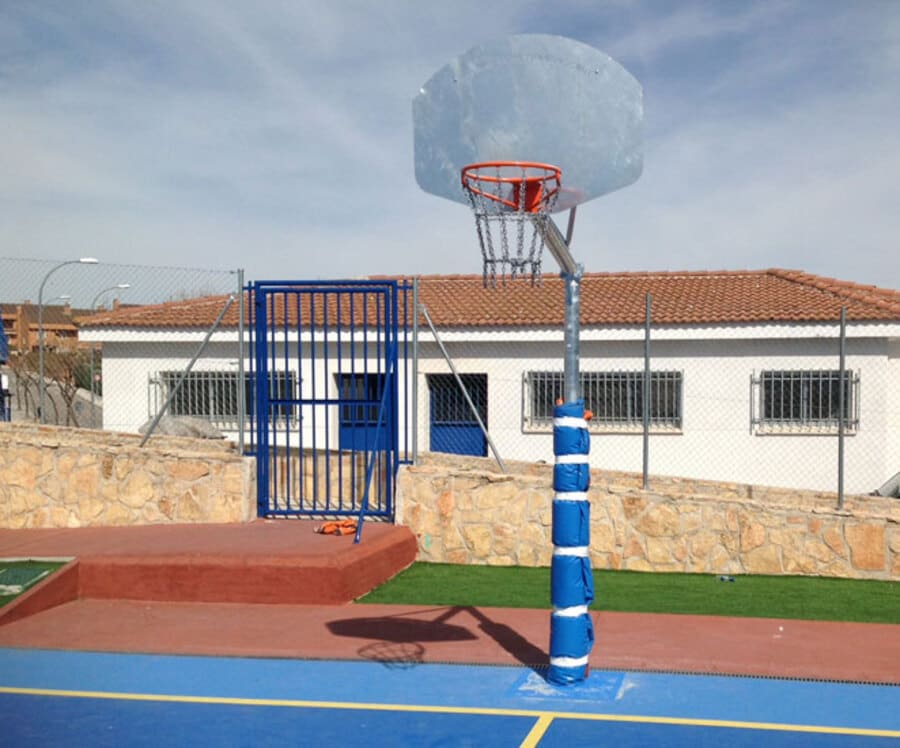The outdoor photograph captures a cloudy day centered around an inviting basketball court. Dominating the middle of the scene is an orange basketball hoop with a sturdy chain net and a solid gray backboard. The hoop's pole is cushioned with a blue mat, secured with white straps, providing safety and a pop of color. The court itself features a striking blue surface marked with yellow lines, enhancing its vibrant appeal. Surrounding the court is a sloping stone walkway, transitioning into a green patch of grass, and bordered by a high chain-link fence. A blue gate door offers entry to the fenced area, suggesting a sense of community access. Beyond the fence stands a white ranch-style building with a brown tiled roof, characterized by three long windows fitted with bars—hinting at either a secure community center or a uniquely-styled home. The overcast sky adds a muted backdrop, emphasizing the mid-day setting with diffused natural light.